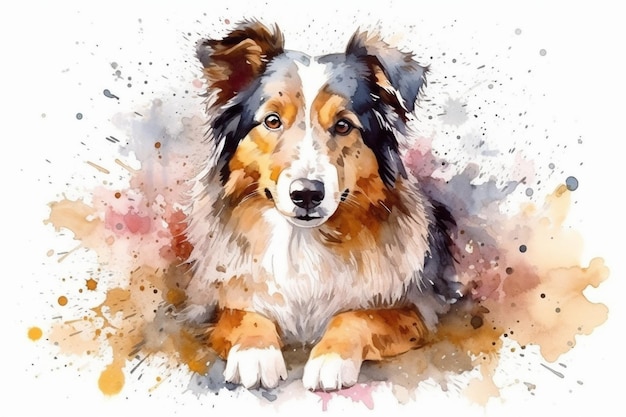This image is a detailed, colorful painting, likely created using traditional or AI technology, depicting a serene and calm dog that appears to be a collie, possibly a border collie. The dog, positioned centrally against a white background, is lying down with its two white-tipped front paws outstretched. The dog's fur is a blend of colors, with a notable pattern: black fur crowns the top of its head and runs down the sides of its face, intersected by a white stripe that leads down to its black nose and forms a straight line up from the muzzle to the top of the head. The face is accented with tan around the eyes and muzzle, while the chest and neck boast long white fur. The calm, closed mouth and round brown eyes of the dog create a gentle expression. Surrounding the dog are splashes of vibrant colors, including pink, orange, red, gray, dark blue, and tan, resembling paint splatters, which add a playful and artistic touch to the composition. The ears, floppy and brown, add to the dog's endearing appearance, completing this harmonious and lively artwork.